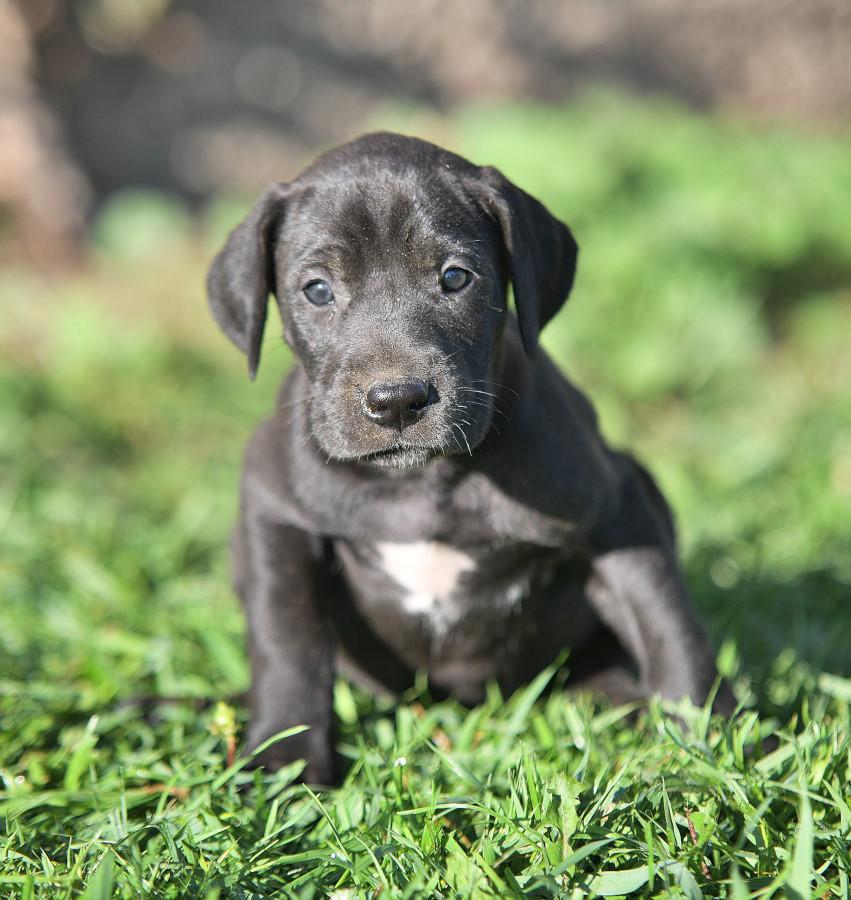This is a nearly square photograph of an adorable, small black puppy with a white splotch on its chest, subtle enough to add to its charm. The puppy, which resembles a black Labrador, has floppy ears that hang down and deeply expressive dark eyes that seem to be steadily gazing at the photographer, hinting at a calm yet curious demeanor. Its short fur is primarily black with the exception of that slight white patch, and its little nose and whiskers are nicely detailed. The image skillfully employs an artistic bokeh effect; the foreground features sharply focused green grass with crisp individual blades, while the middle ground focusing on the puppy's face remains clear, and the background dissolves into a pleasant blur of greens and abstract circles, reflecting the sky. The puppy appears to be in a relaxed, semi-sitting pose, somewhere between sitting and lying down, with its front paws visible. The overall mood of the photograph evokes a warm, inviting feeling, likely to make any viewer want to reach out, pet the puppy, and experience its endearing presence up close.